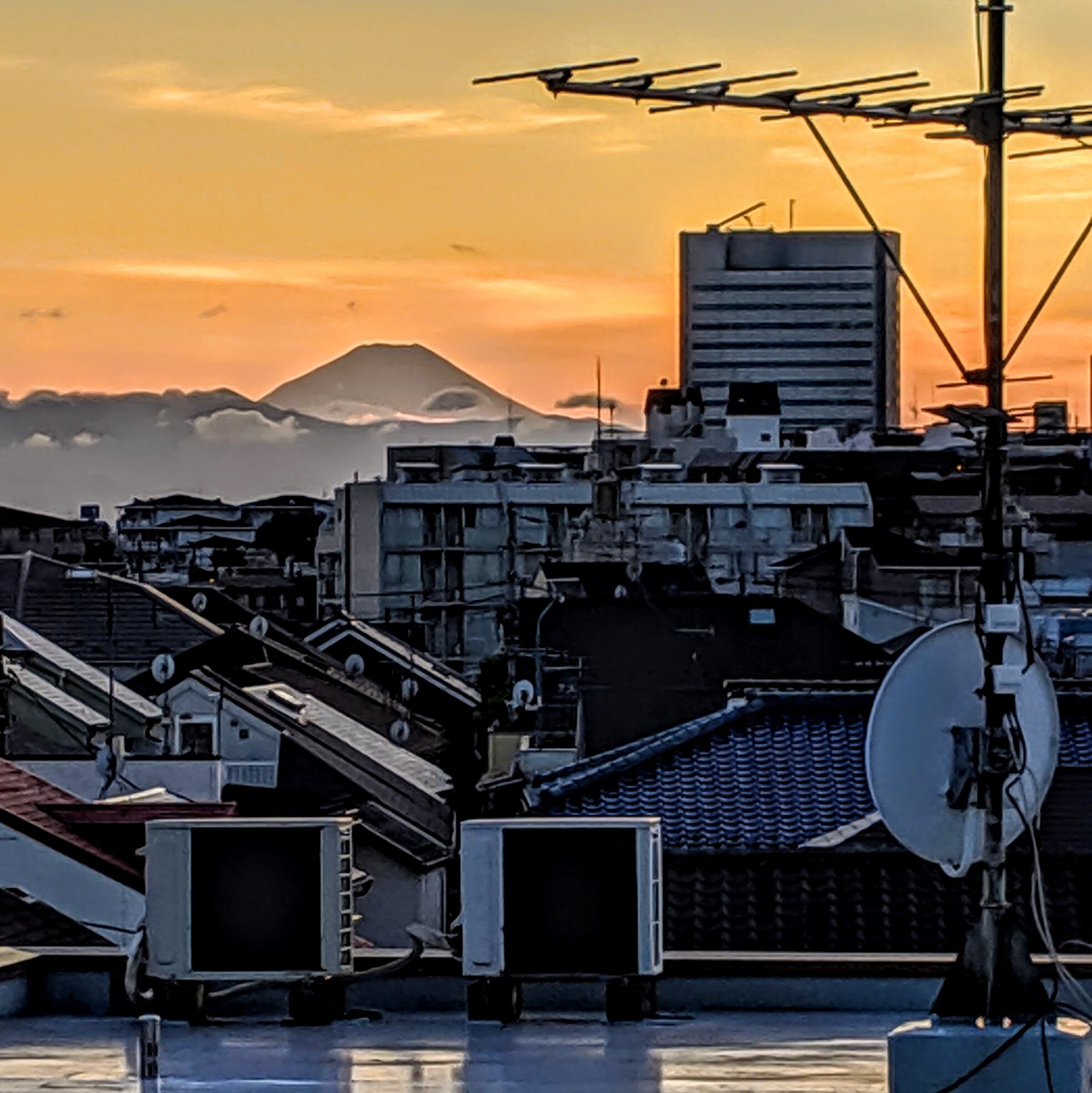The image showcases a vibrant outdoor scene near sunrise or sunset, bathing the sky in a beautiful blend of orange, pink, and peach hues. Wispy clouds scatter across the upper part of the sky, while thicker clouds pile up closer to the horizon. A majestic mountain peak stands prominently in the distance, with dark gray clouds hovering in front, adding a dramatic touch to the landscape. The photograph appears to be taken from a rooftop, evident by the presence of a satellite dish and an antenna on the right. Several other rooftops, equipped with similar dishes and utility units, extend into the background. A slick reflection on one roof suggests recent rain. A towering building dominates the top-right section, featuring multiple structures on its roof, including an antenna and a crane-like apparatus angled against the sky. The scene not only captures the natural beauty of the mountainous background but also the bustling urban elements of rooftops and buildings.